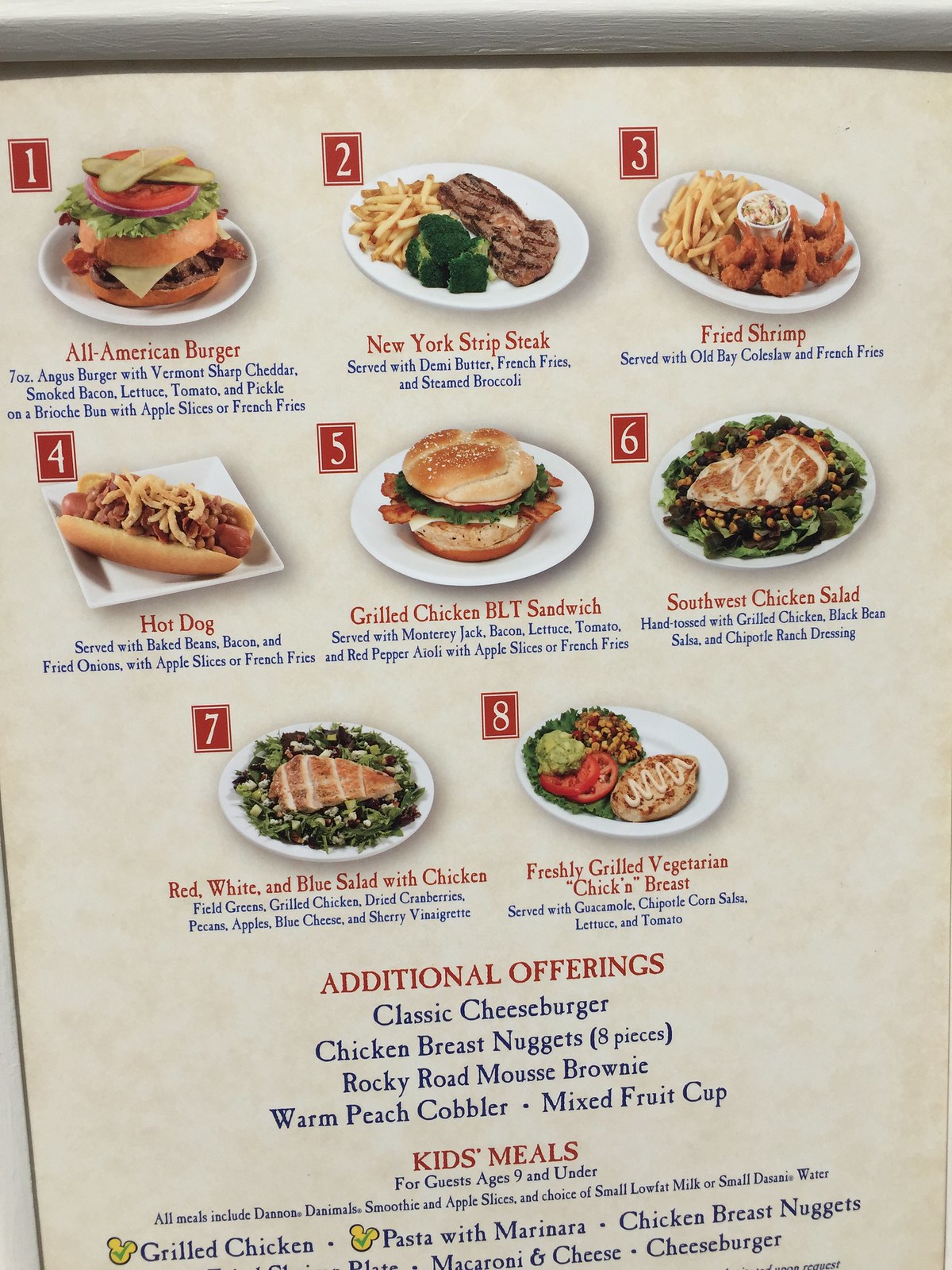**Detailed Menu Description:**

The menu features a distinct pinkish-brown, mingled background and is organized with clear visual elements that make it easy to read.

1. **Top Section**:
   - **Numbering and Color Coding**: Each dish number is highlighted in small red blocks with white numbers, ensuring they stand out. The dish names are written in red, while their descriptions are in blue for clarity.
   - **Dishes**:
     1. **All-American Burger**: A classic favorite highlighted as the first option.
     2. **New York Strip Steak**: A premium steak option, noted for its quality.
     3. **Fried Shrimp**: Presented with a mouthwatering image, making it tempting to seafood lovers.
     4. **Hot Dog**: A simple yet popular choice.
     5. **Grilled Chicken BLT**: A healthier sandwich option.
     6. **Southwest Chicken Salad**: Perfect for those craving a bit of spice.
     7. **Red, White, and Blue Salad with Chicken**: A patriotic-themed, hearty salad.
     8. **Freshly-Grilled Vegetarian Chicken Biscuit**: A thoughtful choice for vegetarian customers.

2. **Additional Offerings**:
   - **Heading in Red**: This section is clearly marked, ensuring customers notice the extra options.
   - **Items in Blue**:
     - **Classic Cheeseburger**: Another traditional favorite.
     - **Chicken Breast Nuggets, Eight-Piece**: Ideal for sharing or a hearty snack.
     - **Rocky Road Mousse Brownie**: An indulgent dessert option.
     - **Warm Peach Cobbler**: Perfect for those who enjoy a comforting dessert.
     - **Mixed Fruit Cup**: A lighter, healthier choice.

3. **Kids' Meals**:
   - **Heading in Red**: Clearly marked for easy identification.
   - **Sub-Heading in Blue**: Specifies that these meals are for guests aged nine and under.
   - **Dishes with Yellow Highlight**:
     - **Grilled Chicken**: A healthy and tasty option.
     - **Pasta with Marinara**: A kid-friendly classic.
     - **Chicken Breast Nuggets**: Always a hit with children.
     - **Macaroni and Cheese**: Comfort food that kids love.
     - **Cheeseburger**: A smaller version of the classic favorite for kids.

This detailed menu ensures all offerings are easily visible and distinguishable, catering to a variety of tastes and preferences.